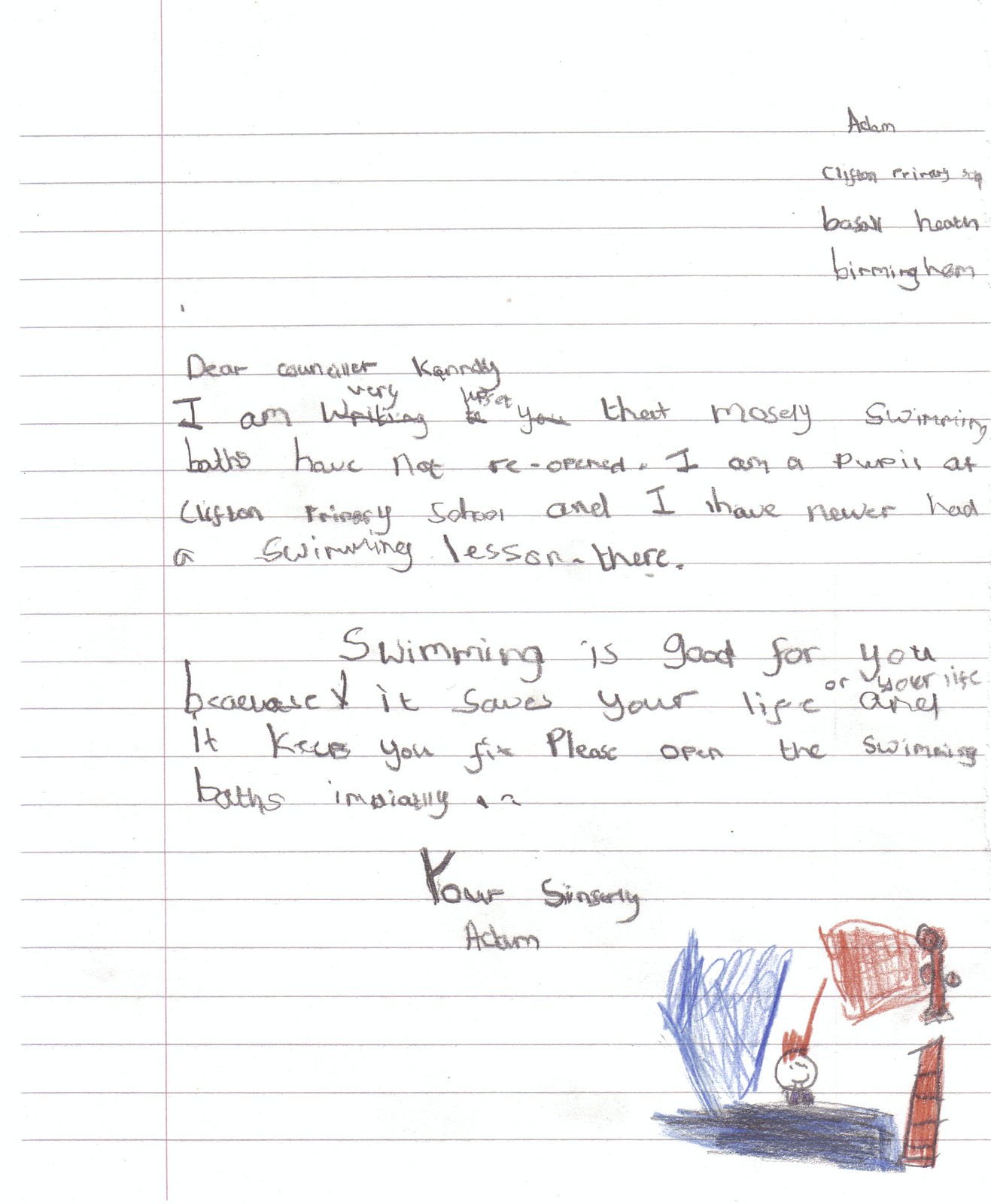The image depicts a scan of a handwritten letter by a child on a piece of white ruled notebook paper, which appears somewhat transparent in the scan. The writing in the top right corner, though very small and difficult to decipher, seems to include the name Adam Clifton and the location Birmingham. Starting on the left, the letter is addressed to a "Councillor Kenny Kennedy" and reads:

"Dear Councillor Kennedy, I am writing to inform you that Mosery Swimming Baths have not reopened. I am a pupil at Clifton Primary School and I have never had a swimming lesson there. Swimming is good for you because it can save your life and keep you fit. Please reopen the swimming baths immediately. Yours sincerely, Adam."

The handwriting is somewhat scribbled and sloppy but mostly legible. The letter includes a child's drawing in the bottom right corner, depicting a boy swimming in what looks like a pool or swimming bath, emphasizing the plea to reopen the swimming facilities.